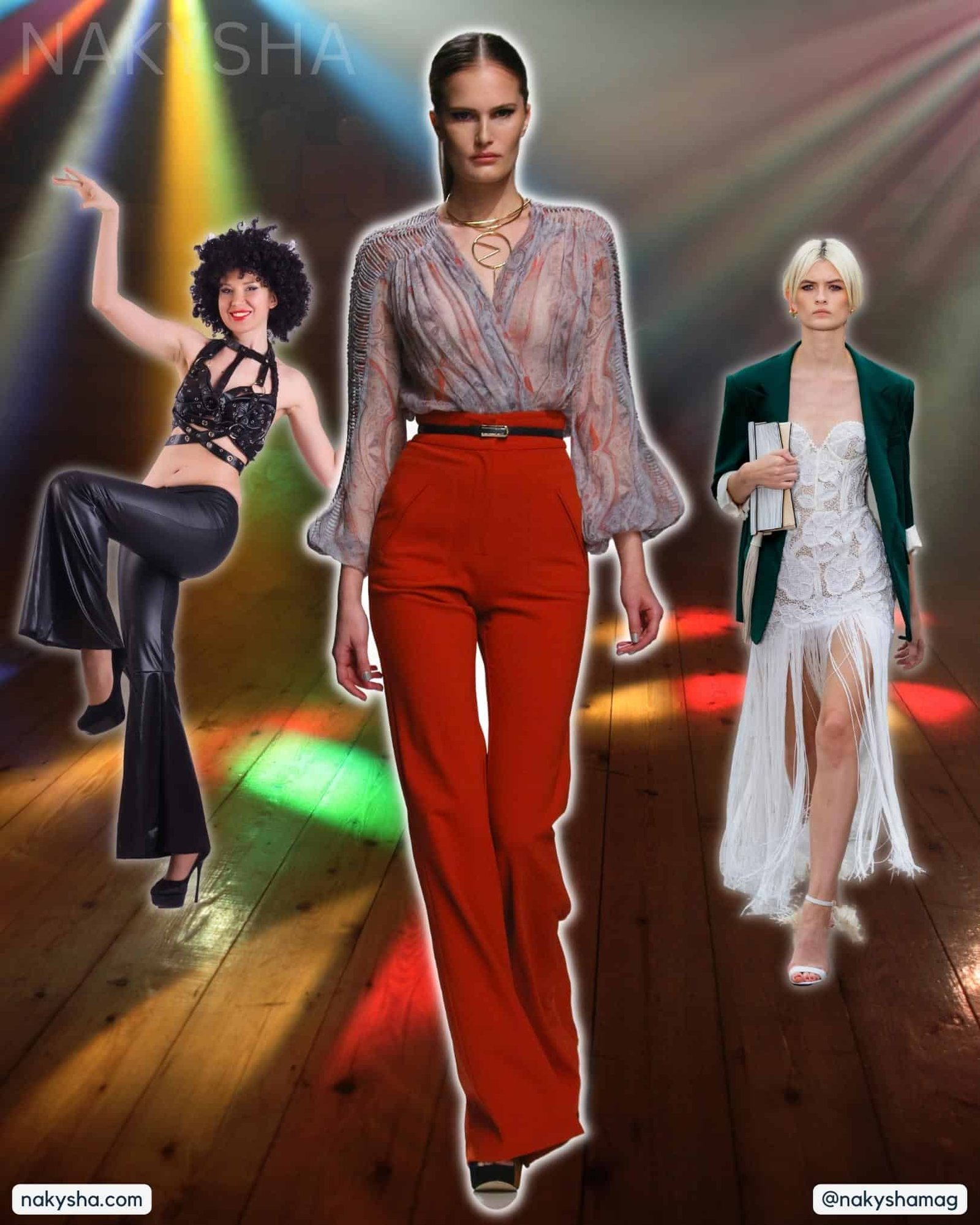The image resembles a web page advertisement featuring three models striding along a wooden platform illuminated by colorful, dramatic lighting, suggestive of a vibrant, artistic composition. At the top left corner, the text "Nakisha" is prominently displayed, while the bottom edges feature the website "nakisha.com" and the handle "@nakishamag."

The model on the left is striking a dynamic pose, sporting a black tank top with metallic accents and revealing leather straps paired with glossy black leather bell-bottom pants. Her towering black high heels elevate her look, while her voluminous, curly black hair adds a theatrical flair. Purple, red, cyan, white, and blue lights cast an effervescent glow around her.

At the center, another model is confidently walking forward in red pants cinched at the waist by a black belt with a brass buckle. She wears a sheer, frilly blouse that transitions in hues from pink to purple to blue, complemented by a gold chain necklace with a significant pendant. Her brown hair, pulled back in a ponytail, frames her stern expression.

To the right, the third model exudes a sophisticated vibe in a white lace dress with a flowing, stringy skirt, paired with a green blazer draped over her shoulders. Her white sandals peek through as she holds a clutch in her left hand. Her blonde hair, tied back and parted in the middle, together with her light-colored skin, harmonizes with the white and green lights enveloping her. 

Rainbow-colored beams illuminate the wooden floor, contributing to a surreal ambiance that contrasts with the models' poised, runway-ready stances, suggesting an intricate blend of photography and digital artistry.